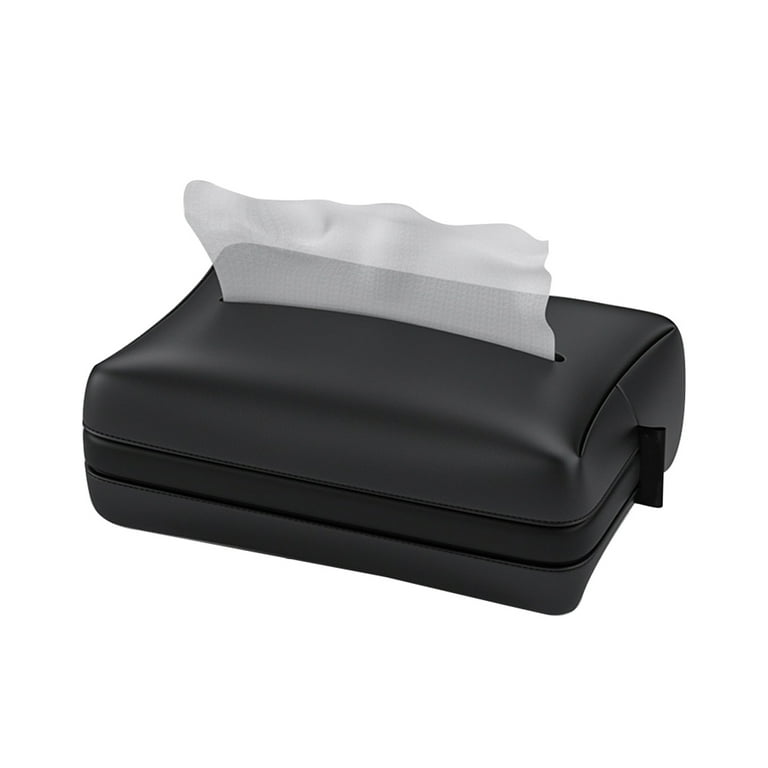The image features a close-up of a sleek, black tissue holder, predominantly made of a smooth, leather-like material with plastic elements. The holder is designed with a soft-touch appearance and smooth, curved edges that add to its cushion-like look. Positioned slightly at an angle, facing downwards to the left, the black tissue holder prominently displays a single white, semi-transparent tissue emerging from a slit at the top. The tissue appears delicate with a faintly woven texture. To the right of the holder, there's a small rectangular black tag attached to it. This detailed image of the tissue holder is set against a plain white background, devoid of any other objects or branding, creating a simple and clutter-free composition. The lighting is bright and clear, accentuating the textures and details of the holder and the tissue.